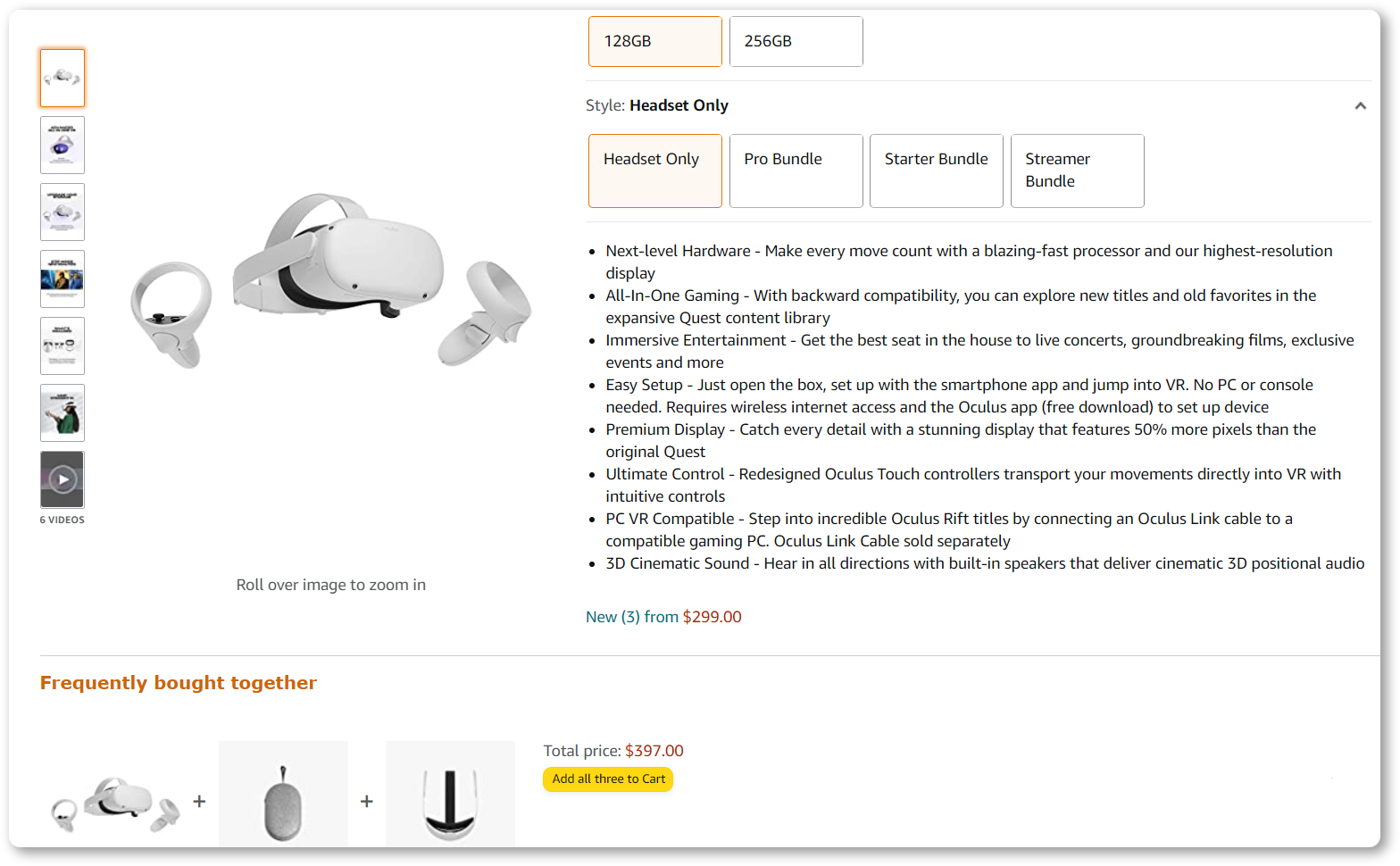**Detailed Caption:**

This image is a screenshot of an Amazon product page showcasing a VR headset. On the left side of the screenshot is a high-resolution photo of the VR headset. On the right, there are two buttons at the top for selecting different memory sizes: "128 GB" and "256 GB." The "128 GB" option is highlighted in gold, indicating it is currently selected, while the "256 GB" option has a black outline against a white background.

Below this, there is a section titled "Style" with four clickable options, each represented as buttons: "Headset Only," "Pro Bundle," "Starter Bundle," and "Streamer Bundle." The "Headset Only" option is highlighted in gold, signifying it's the selected choice.

Further down, a bullet-point list elaborates on the key features of the VR headset:
- **Next-Level Hardware:** Experience every action with a blazing-fast processor and the highest resolution display.
- **All-in-One Gaming:** With backward compatibility, users can explore both new titles and old favorites within the extensive Quest content library.
- **Immersive Entertainment:** Enjoy front-row seats to live concerts and other immersive experiences.

This organized layout provides a comprehensive overview of the product's specifications and bundled options, helping users make informed decisions.